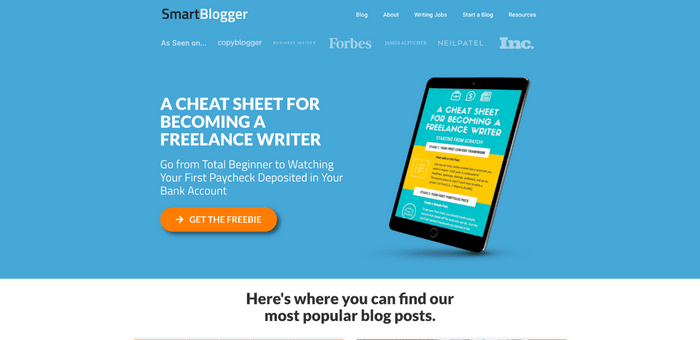The advertisement features a predominantly blue background with the word "Smart" in black at the top, followed by "Blogger" in white. The remainder of the text is also in white, though much of it appears blurry, mentioning topics such as wanting jobs, starting a blog, and various resources. 

Prominently, the ad notes endorsements from sources like Copyblogger, Forbes, and Inc. To the right side of the ad, there is an image of a black tablet. The tablet’s screen displays a blue background with the text "A Cheat Sheet for Becoming a Freelance Writer." Below this main text, additional smaller text provides further description about the cheat sheet, which helps individuals go from complete beginners to receiving their first paychecks from freelance writing.

An orange oval-shaped button below the text on the tablet reads "Get the Freebie" in white letters. The bottom part of the ad has a white background with black text that says, "Here is where you can find our most popular blog posts."